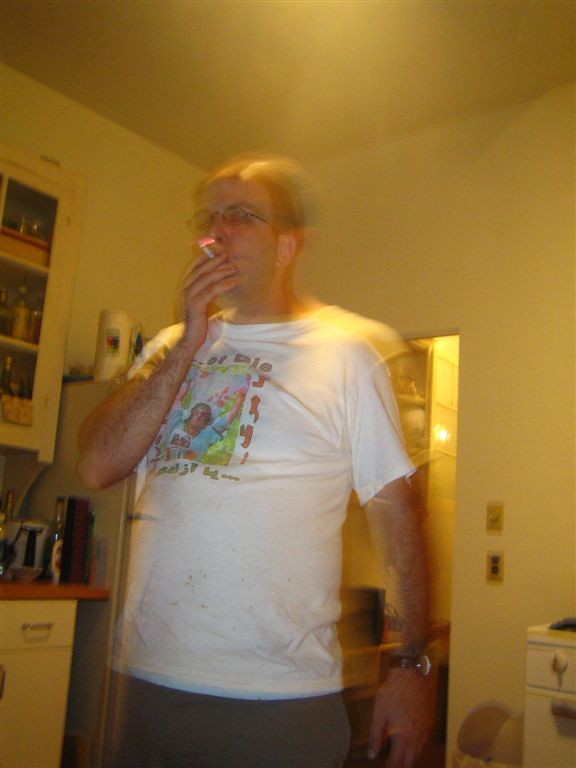A middle-aged man, approximately 45 years old, stands in his kitchen, cigarette in hand. He is taking a drag and appears to be savoring the moment. Dressed in a white T-shirt with the partial slogan "or die" visible, the shirt has an image of a man who resembles Jack Black having a wild time. He also sports a pair of glasses, a watch, and is wearing grayish-brown khaki shorts. The kitchen setting is evident from the refrigerator behind him and a stove to his right, with various items on the shelves adding to the domestic scene. Light from above highlights the smoke-filled room, suggesting this is likely his second cigarette. The image captures a blend of humor and casual demeanor, with the man’s relaxed posture adding to the snapshot of everyday life.